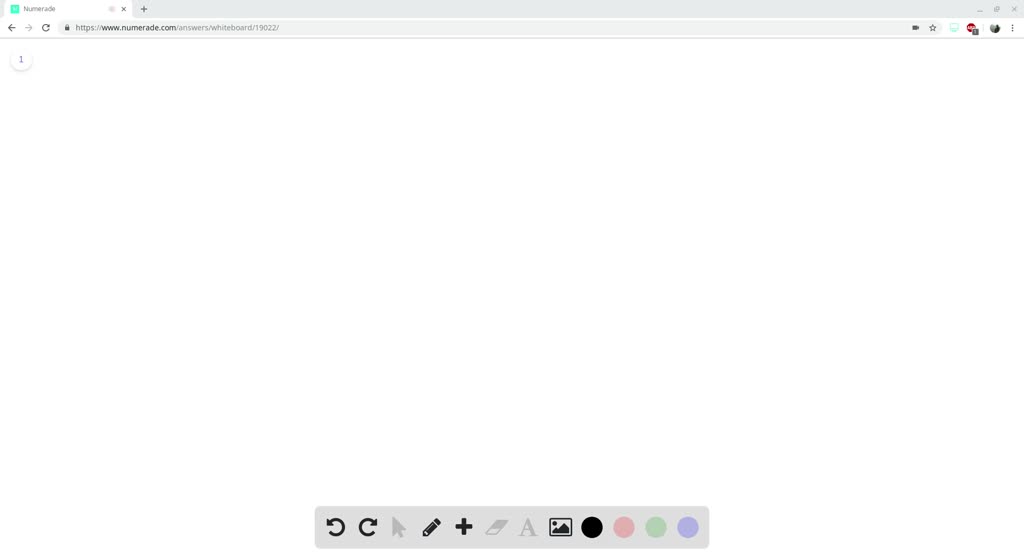The image showcases a screenshot of a software interface, likely a web browser, judging by the presence of a refresh button and a back arrow typically found in such applications. Though the URL is visible, it is too small to decipher. The main portion of the screen is blank and white, indicating an empty or loading workspace. Below this area, there is a toolbar featuring several icons: an undo button, a redo button, a pencil tool, a plus sign, and an image insertion button. Additionally, there is a black circle icon, possibly indicating the color of the pencil tool, suggesting that drawing with the pencil will produce a black line.